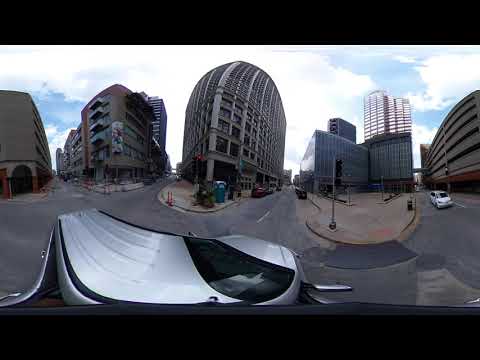The image appears to be taken with a fisheye or 360-degree lens, creating a rounded and immersive view of a dense city block. Central to the scene is a large office building, approximately 12 to 14 stories tall. Flanking this main building are several other structures, including a notable corner building with distinctive porches or decks extending outward over the street, giving a residential feel. To the left, a third building peeks into view, partially cropped out. The streets are narrow and intertwine closely between the buildings, suggesting an older urban design, perhaps reminiscent of European cities like those in Italy. Among the details, there's a white car moving towards the camera, multiple empty streets, parking garages, and a solar-paneled vehicle. Cones and a port-a-potty indicate ongoing road construction. The sky is a clear blue with scattered white clouds, emphasizing the sunny, pleasant weather. The scene, bustling with architectural and urban detail, offers a unique and condensed view of city life.